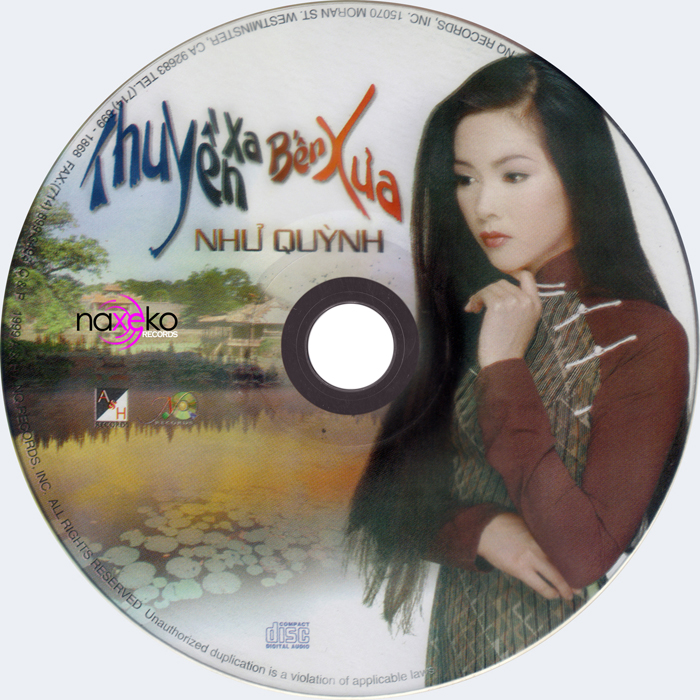This music CD, titled "Thuynh Binh Nhua" with the subtitle "Nu Khunya" in bronze, features an image of an Asian woman on the right-hand side. She has long black hair cascading down to her waist and is dressed in a rust-colored long-sleeve shirt with a tan brown top adorned with white strings, resembling a Japanese-style kimono. The woman is captured in a contemplative pose, looking towards the left with one arm resting across her waist and her left hand touching her chin. The background of the image showcases a serene pond with lily pads, a small wooden house, and some trees, while the remaining background outside the disc is a soft white. The CD also has the words "Thuyen" in blue, "Zaben" in green and orange, and "Zua" in orange inscribed on it. The address "Westminster, California" indicates its production in the United States, though some of the text appears to be in a language other than English.